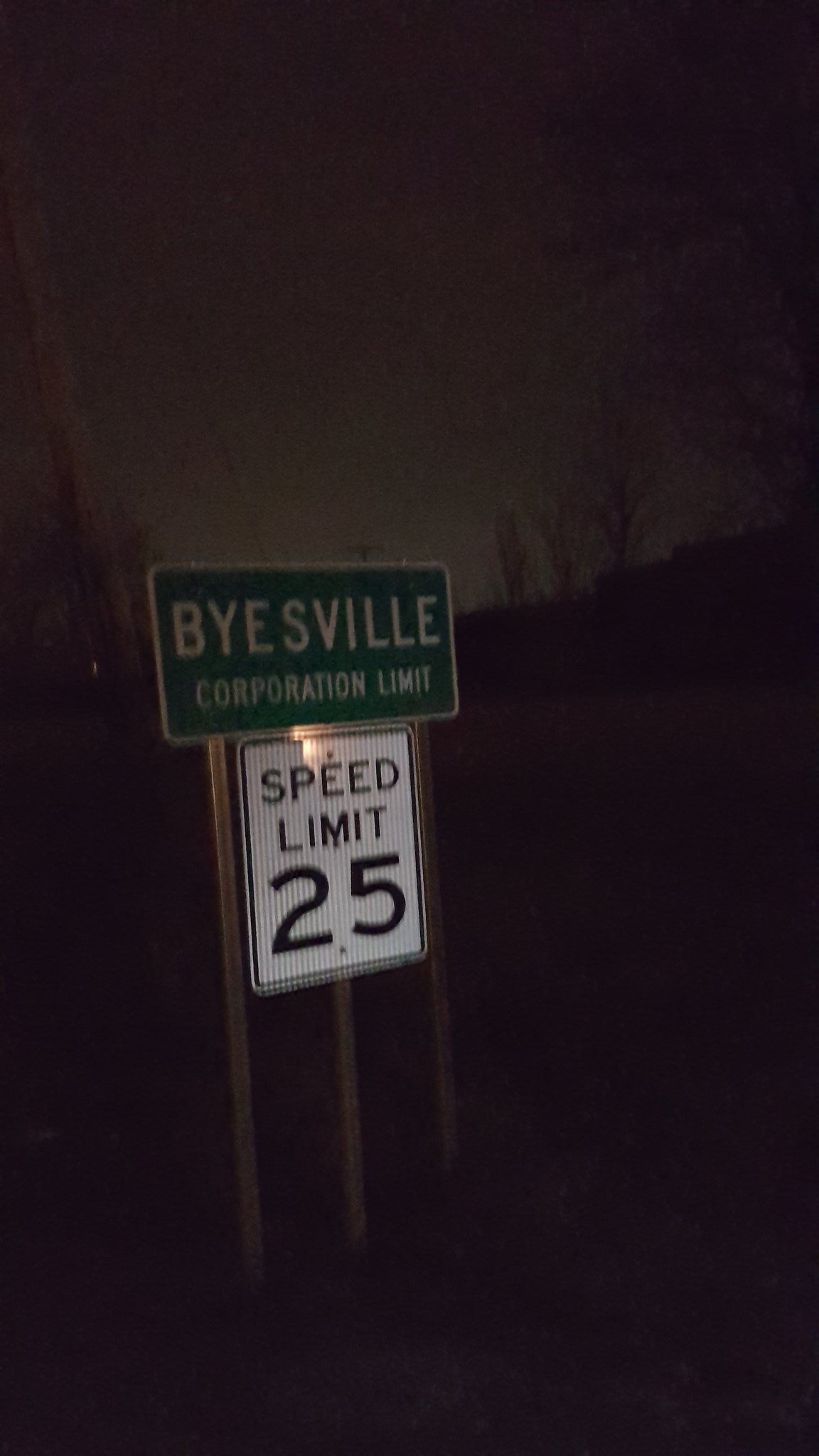This atmospheric nighttime photograph captures a dark outdoor scene. The focal point is a road sign anchored by three metal bars that descend into the ground. The bottom sign is white, bordered in black, and displays "Speed Limit 25" in bold, black lettering. Just above it, there is a green sign with a white border and text reading "Buysville Corporation Limit." The backdrop features a dimly lit area above the signs, likely illuminated by a distant light source, adding a faint glow to the surroundings. This light subtly highlights the outlines of tree branches against the dark night sky, while the ground below remains shrouded in darkness, emphasizing the solitude and quiet of the scene.